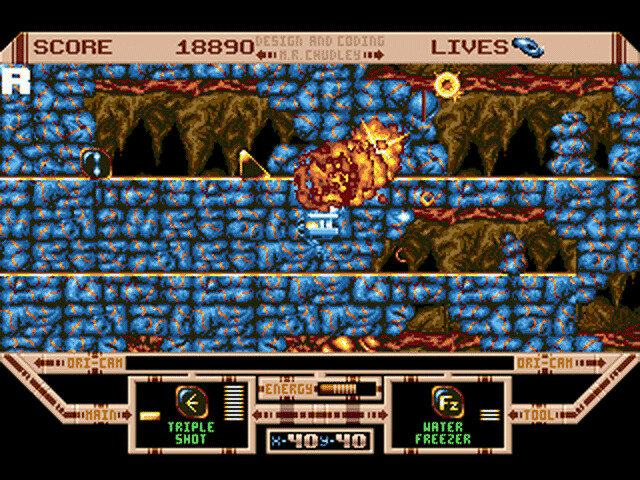In this screenshot of a retro-style video game, the display features a classic black-bordered background at both the top and bottom. At the top section, an off-white, tan-colored stripe with brownish-red text reads "SCORE 18890" and "LIVES," accompanied by a blue icon. Additionally, in grey print, the text "Design Encoding M.R.Chudley" is visible. 

The main game area showcases a blue, rocky-textured background interspersed with orange veining, giving the scene a vibrant yet rugged appearance. At the center of the screen, an orange-colored explosion stands out dramatically against the rocky terrain. 

To the lower portion of the screen, detailed HUD elements are displayed. On the left, an icon labeled "Triple Shot" features a left-pointed arrow. Next to it, indicators labeled X and Y both display the number 40. An energy bar, situated nearby, is half-full, showing the player's current energy level. Lastly, an icon marked “FZ” with the label “Water Freezer” is also visible.